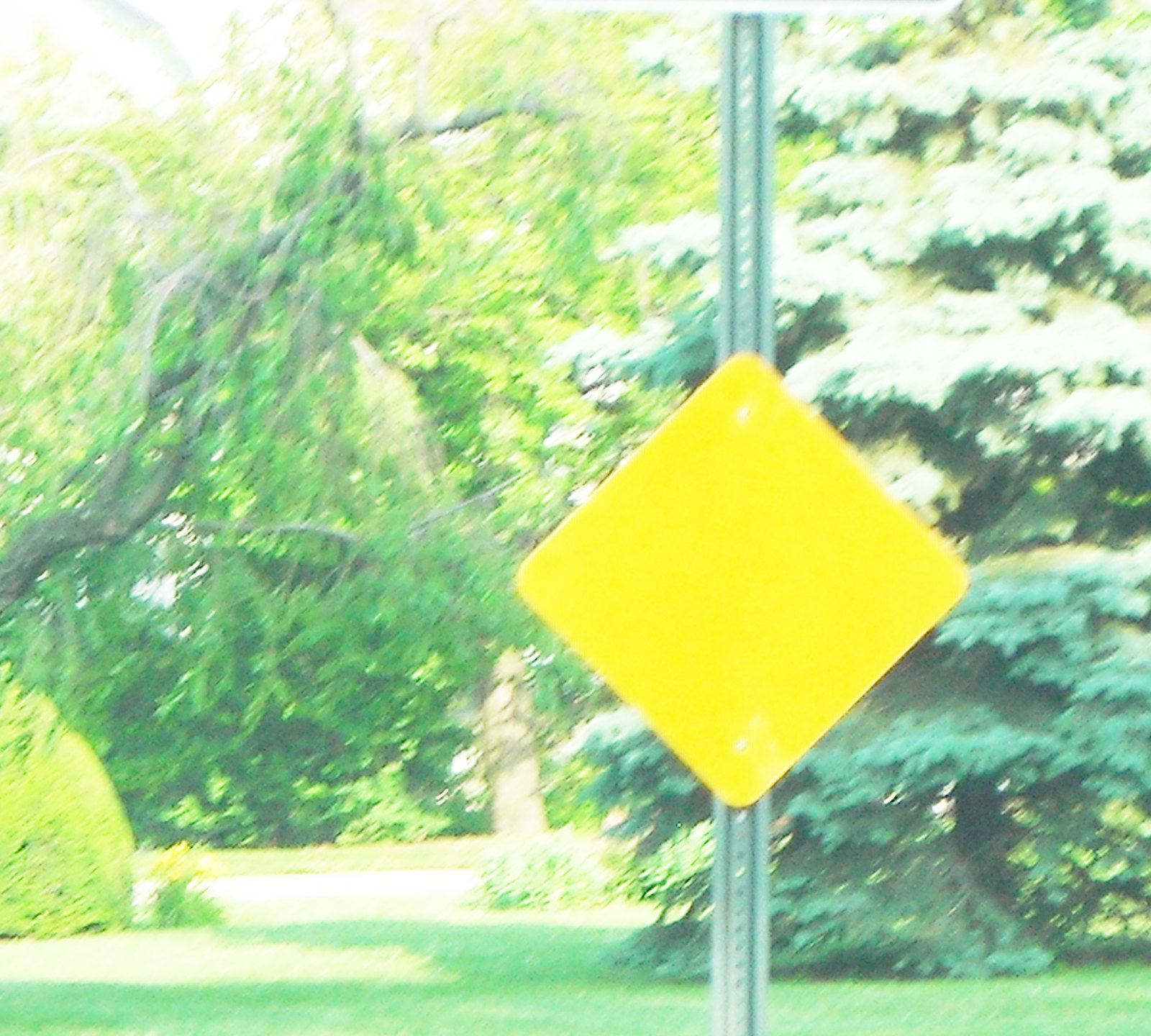In the foreground of the image, a prominent diamond-shaped yellow sign is affixed to a tall metal pole punctuated with numerous holes, hinting at its adjustable mounting system. The pole stands on a grassy expanse, with the ground covered in fawn-colored grass. To the left, the grass transitions into a lush green, while on the right, a green tree with vineyard-like leaves adds depth to the scene. In the distant background, a majestic willow tree stands, its extensive and large branches spreading out, with a multitude of smaller branches cascading down, partially obscuring the rear of the image. The entire scene is bathed in bright, vivid light, highlighting every detail with remarkable clarity.